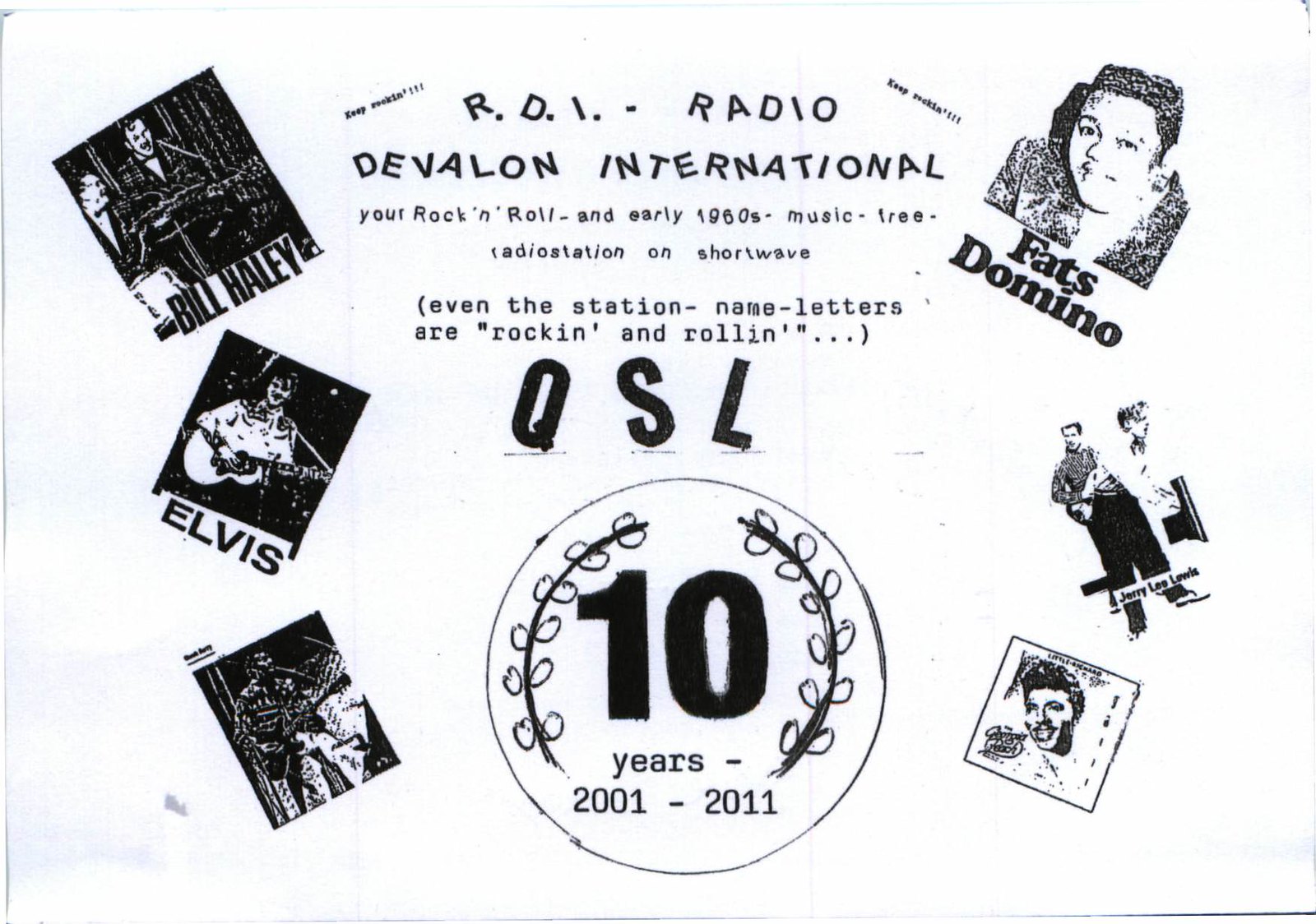The image is a close-up of a black-and-white flyer for a radio station, styled in a vintage design. At the top, bold letters read "RDI Radio," followed by "Devalon International." Beneath that, the text states, "Your rock and roll and early 1960s music free radio station on Short Wave," with the letters "QSL" prominently displayed, appearing to rock and roll. The center of the flyer features a circular logo with laurel branches encircling the number "10," and the years "2001-2011." Flanking the central text are six black-and-white photos; on the left side, the top photo is labeled "Bill Haley," below it is a photo of Elvis Presley, and further down is a photo of an unidentified man. On the right side, the top photo is labeled "Fats Domino," followed by two unlabeled photos, the bottom one appearing to be an album cover of Elvis Presley. The entire flyer exudes the essence of a nostalgic advertisement celebrating a decade of rock and roll music broadcasting.